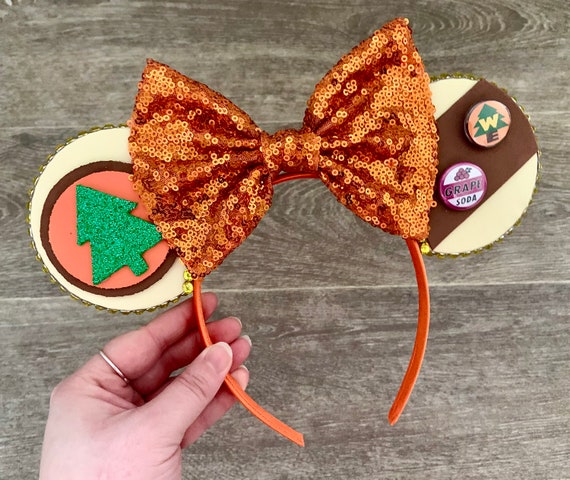In the photograph, a hand with a ring on the forefinger holds an orange plastic headband adorned with a large sequined, dark orange glitter bow in a bowtie shape. The background features gray, driftwood-colored planks, suggesting a tabletop or flooring. The bow is held between the woman's thumb and four outstretched fingers, revealing two decorative, round objects attached to the headband. On the left side of the bow, there's a round piece with a red circle and a brown edge, featuring a glittery Christmas tree cutout in the center. On the right side, there's another round object with a brown stripe, displaying two buttons and resembling a campaign button. The overall look suggests a Mickey Mouse-styled accessory, designed to be secured on the head with a clip. The intricate details and festive decorations hint at a unique, holiday-themed headband.